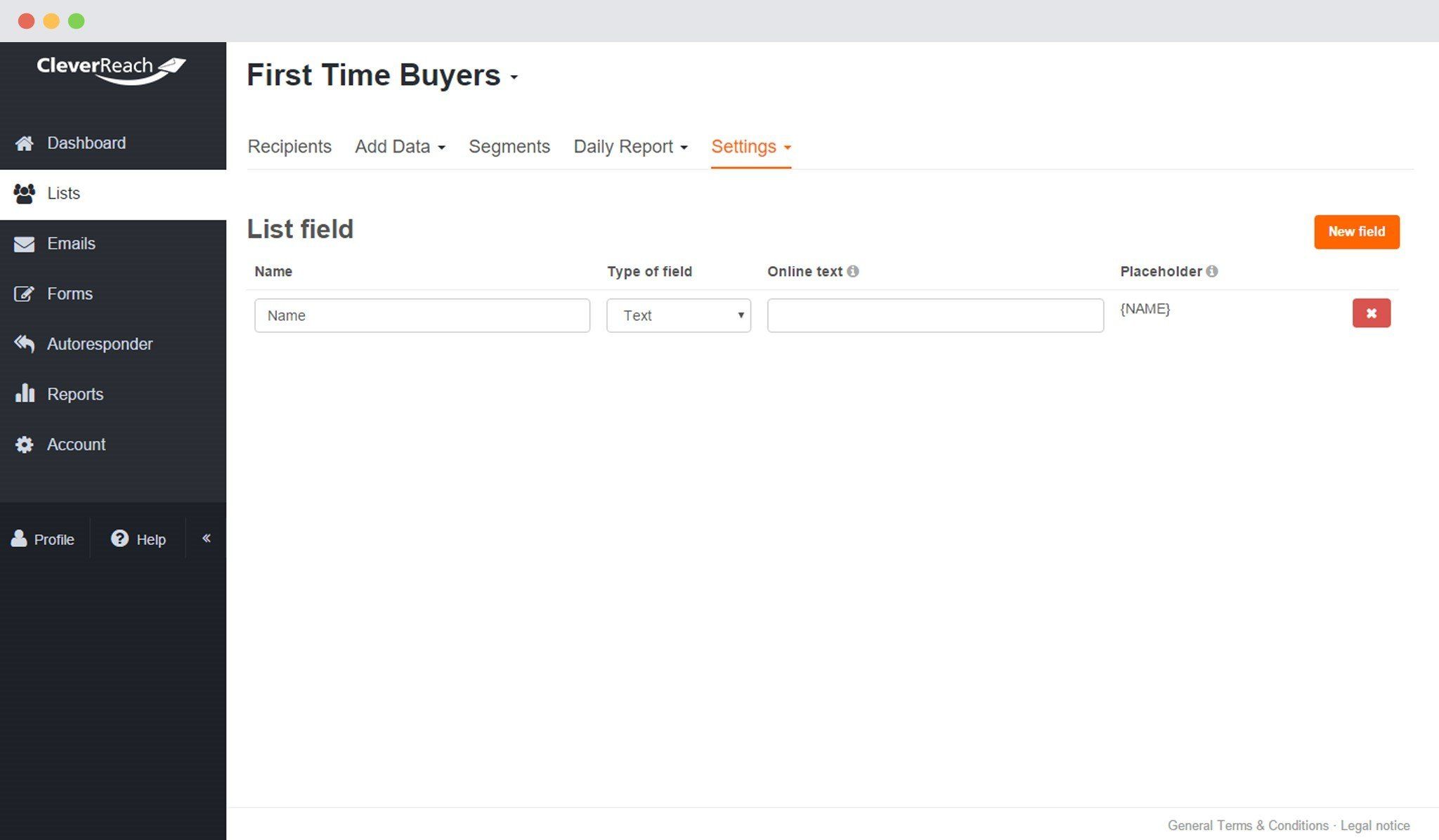This is a screenshot from the Clever Reach section of my website. On the left side of the image, three colored dots—a red dot, an orange dot, and a green dot—are visible, possibly indicating status or progress. To the right, there is a header labeled "First Time Buyers," followed by several navigation options: "Recipients," "Add Data," "Segments," "Daily Reports," and "Settings" highlighted in orange.

Below these options, the "List Field" section is presented. It includes an input field labeled "Name" with a corresponding text box for entry. The type of field is specified as "Online Text," and there is a placeholder text hinting at what should be entered. At the bottom right of this section, a button labeled "New Field" is visible.

Additionally, a white X inside a red square, presumably a close button, is present. On the left side of the screen, there is a vertical navigation menu offering links to "Dashboard," "Lists," "Emails," "Forms," "Founder," "Reports," "Accounts," and "Profile." There is also a "Help" link accompanied by a question mark icon, providing users with assistance.